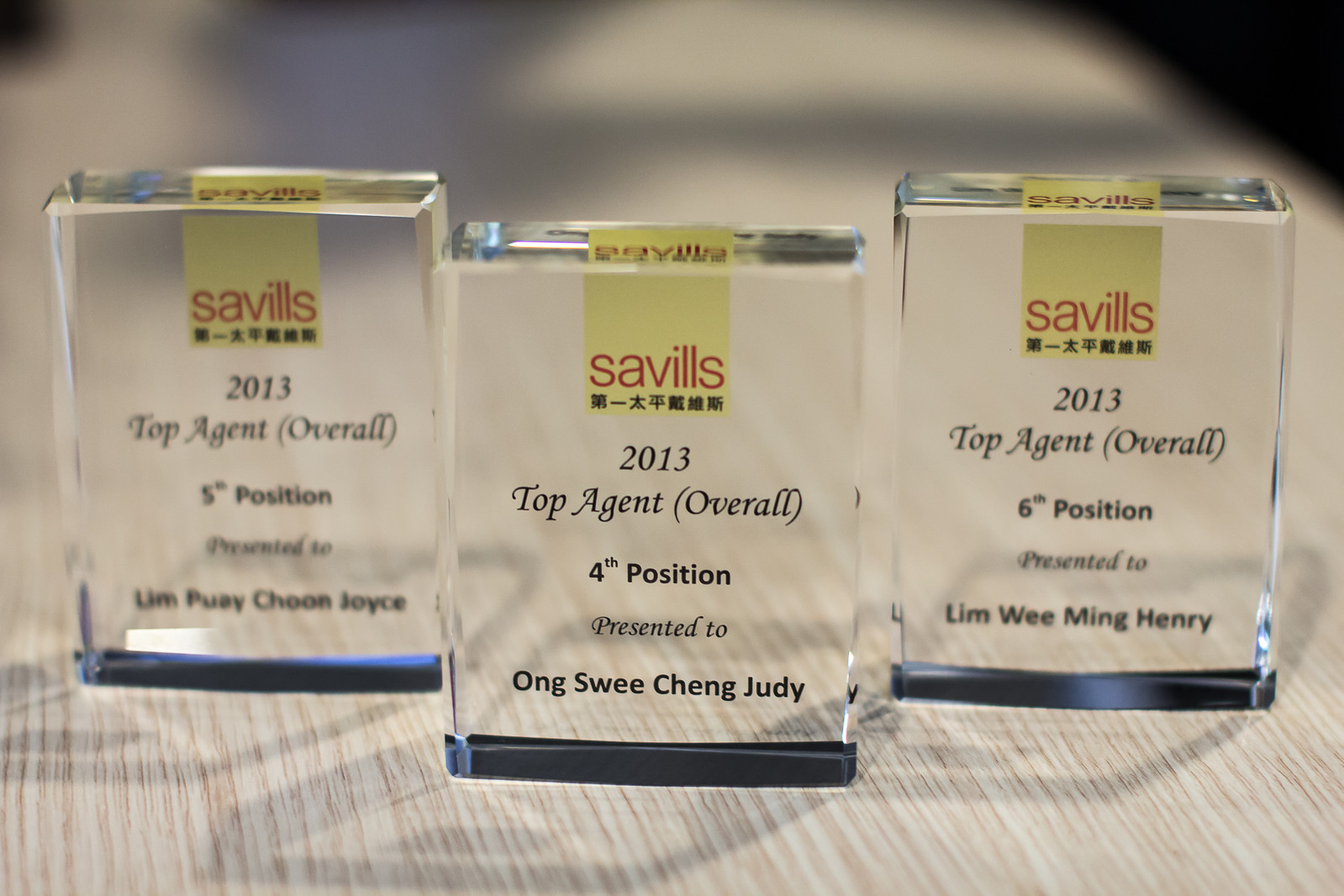This image showcases three elegant, rectangular awards made of clear glass or plastic with black bases, all arranged on a light brown wooden table with visible wood grain. These trophies, presented by Savills, have a distinctive design featuring a yellow rectangular bar at the top with "Savills" in red letters and Chinese characters beneath. All three awards honor the Top Agent Overall for 2013, with each specifying a different position: the leftmost award for 5th position, presented to Lim Pai Chu Joyce; the middle for 4th position, presented to Aung Swee Chan Judy; and the rightmost for 6th position, presented to Lim Wee Ming Henry. The awards are meticulously detailed with consistent inscriptions in black bolded letters, adding to their prestigious and sophisticated appearance.